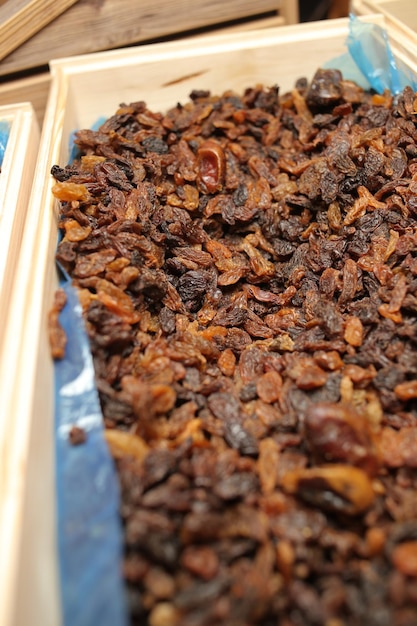This photograph features a wooden rectangular box lined with a blue plastic sheet. The box is filled to the brim with a variety of dehydrated food items, likely dried fruits such as raisins, chili peppers, or sun-dried tomatoes. The contents display a range of colors—some nearly black, some golden, some reddish, and some brown or yellowish-orange, indicating a high degree of dehydration. The box appears next to another similar box, which is partially visible. The use of the plastic lining inside the wooden box suggests it is meant to prevent staining and maintain cleanliness, likely to store and possibly sell these dried items. This visually rich assortment highlights the different stages and types of dehydration among the fruits.